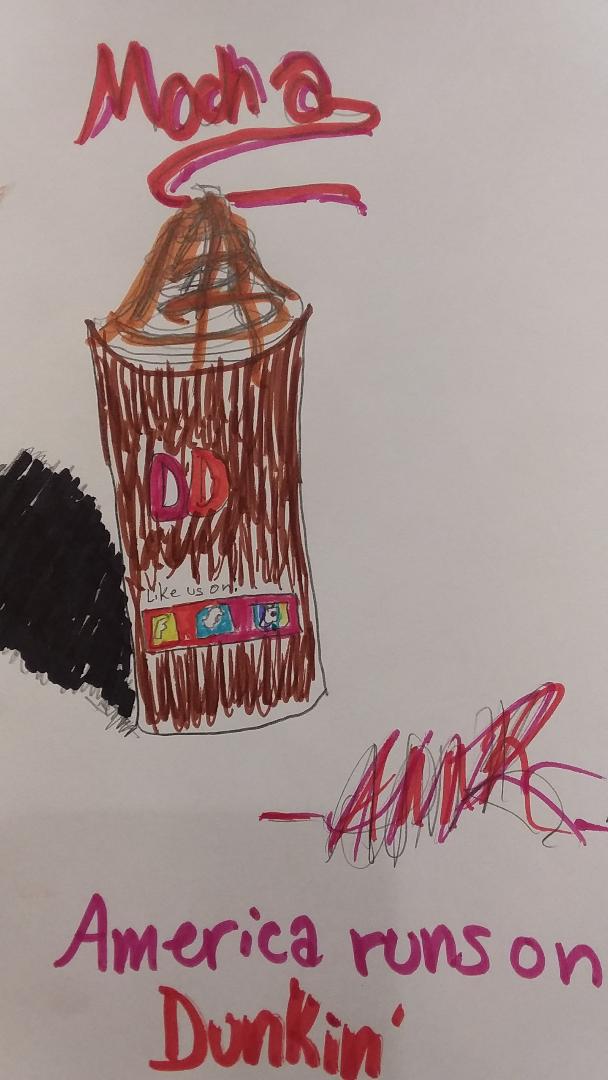This image is a detailed marker drawing of a Dunkin' Donuts coffee cup against a vertical, rectangular white background. At the top of the page, the word "Mocha" is prominently featured in pink and orange lettering with a swirling line descending from the letter 'A'. The central focus is a large depiction of a Dunkin' Donuts cup with a pointed dome lid, embellished with brown lines to represent the coffee within. The cup showcases the "DD" logo in vibrant orange and purple, accompanied by a mix of pink, turquoise, and yellow decorative circles near the lower section of the cup. A horizontal label near the bottom of the cup reads "Like Us On" alongside the symbols for Facebook, Twitter, and Instagram. Below the cup, the slogan "America runs on Dunkin'" is inscribed in purple and orange. Above the slogan, there appears to be a barely legible signature or initials, possibly "AMR".